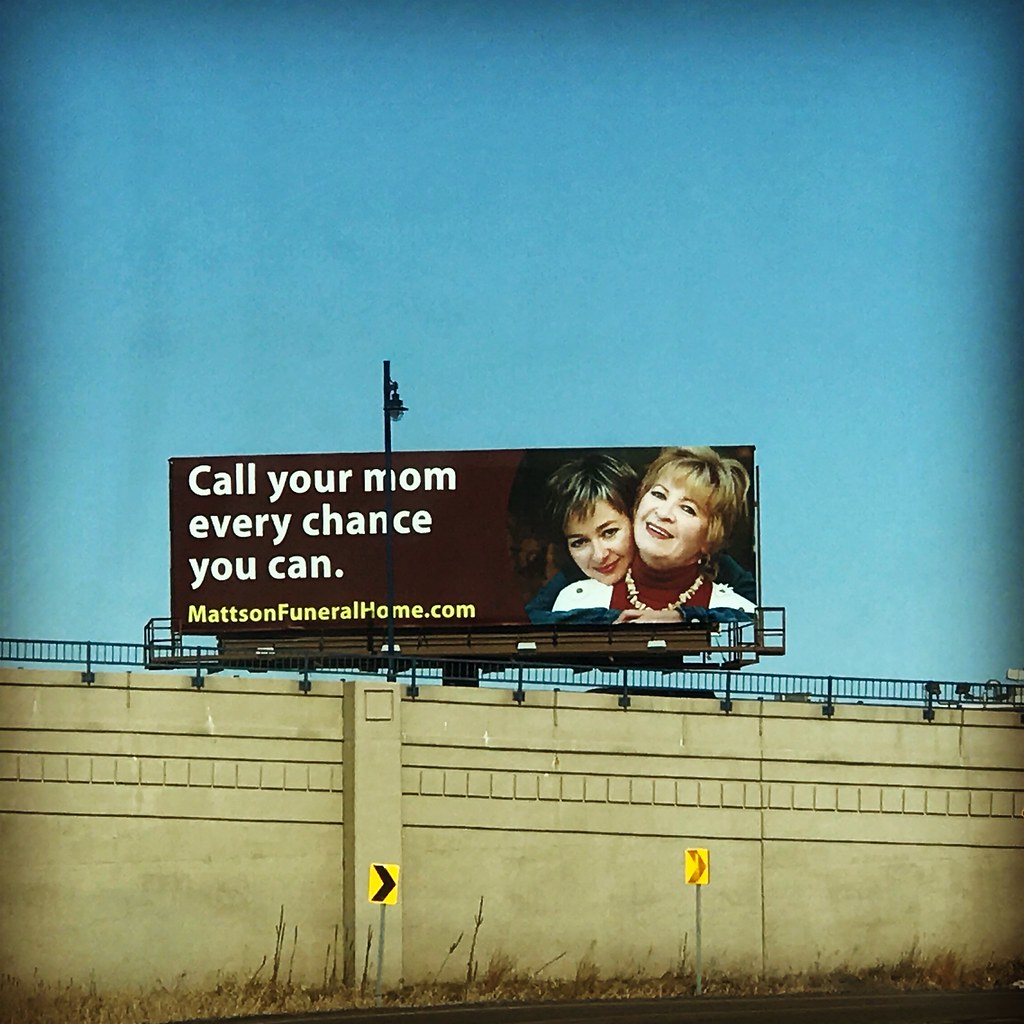This outdoor image, bathed in clear blue skies, captures a concrete overpass with black metal guardrails at the top. Centered within the frame, a purple billboard commands attention with a poignant message: "Call your mom every chance you can." Below this heartfelt reminder, "MattsonFuneralHome.com," is displayed in yellow letters. The right side of the billboard features a touching photograph of an older woman in her early 60s, smiling warmly at the camera, as a younger woman hugs her from behind. In front of the concrete wall guarding the overpass, a grassy area is adorned with two yellow road signs pointing to the right, hinting at a nearby on-ramp leading up to the main road. Light poles and a collection of square concrete shapes add to the urban setting of this evocative and detailed scene.